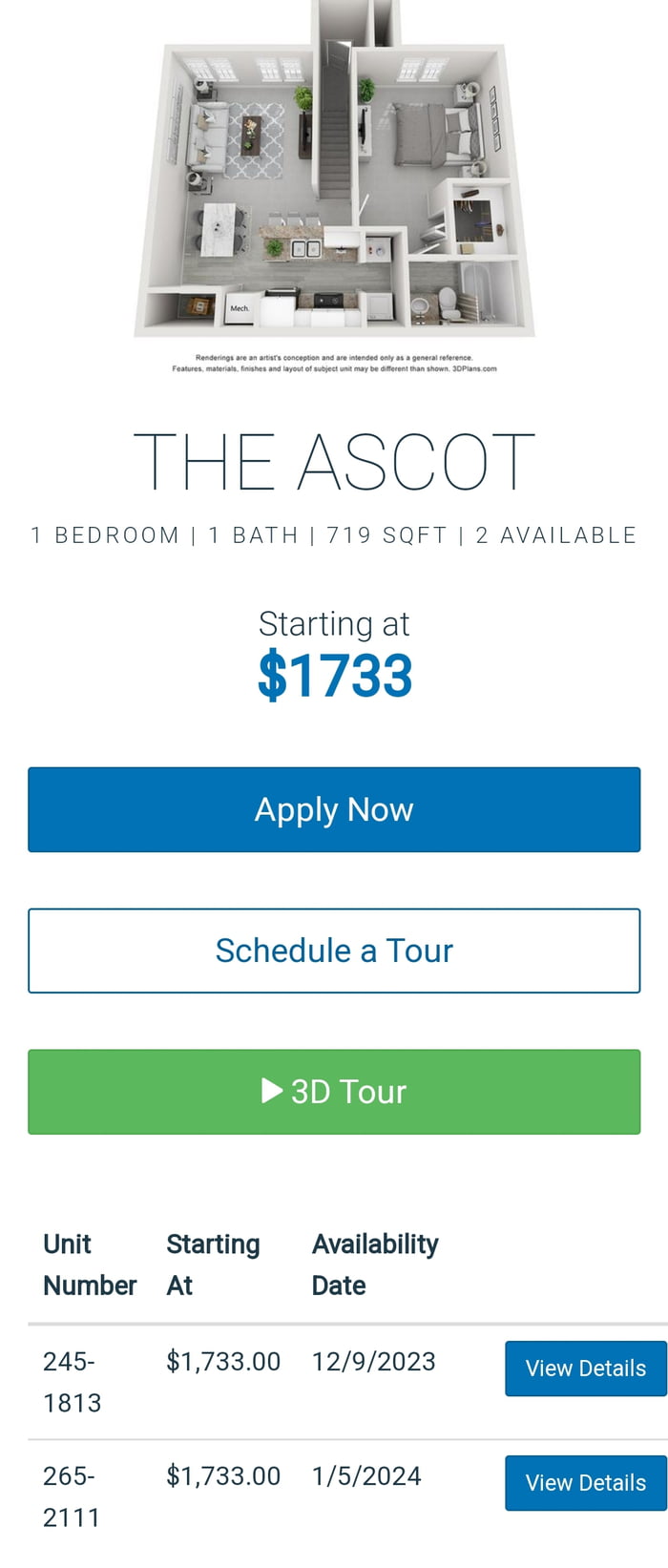This image is a screenshot featuring an available apartment for rent, characterized by its vertical layout, likely indicating it was cropped from a larger webpage rather than a phone screenshot. The background is stark white, creating a minimalist look. At the top of the image, a bird's-eye view of the apartment layout is presented in a detailed 3D render, complete with various pieces of furniture as if currently inhabited.

Directly beneath the 3D model, there are a few sentences of text, though they are not legible. Below this text is the title "The Ascot" in prominent, large font. Accompanying this, it specifies the apartment details: "One bedroom, one bath, 719 square feet, two available." The starting price is clearly marked at $1,733 in a distinct blue font.

Below the pricing information, the image features several actionable buttons: a blue "Apply Now" button, a white "Schedule a Tour" button, and a green "3D Tour" button, intended to engage prospective renters. Further details about unit availability are listed, such as unit number 2451813 available at the price of $1,733 from December 9, 2023, with a corresponding blue button to "View Details." Another unit, numbered 2652111, starts at the same price and is available from January 5, 2024, also featuring a blue "View Details" button.